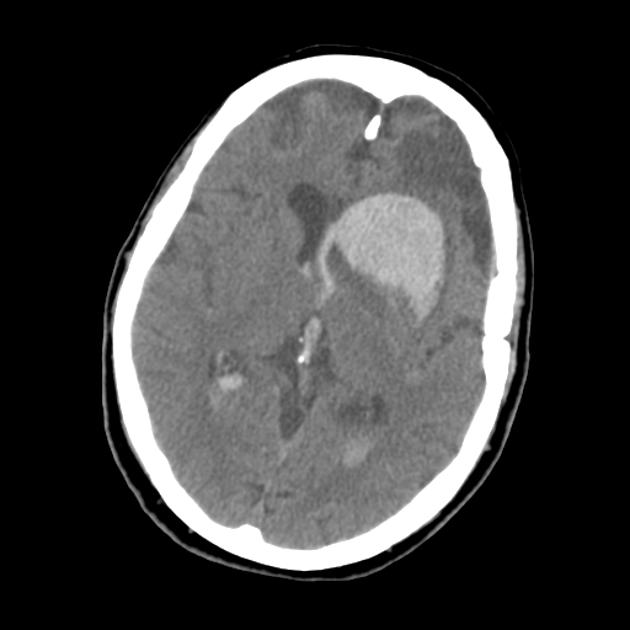This image is an MRI scan of a human brain depicted in black, white, and gray tones, centered with a black background. The scan shows a rounded oval shape representing the skull, characterized by a thin white line contouring the outer perimeter. Inside, a thicker white border indicates the cerebrospinal fluid space surrounding the brain. The brain tissue appears in dark gray shades with notable features including black and white splotches. At the forefront, on the right side, there is a prominent light gray area resembling a ball, likely indicative of an intracerebral hemorrhage, suggesting a collection of blood within the brain tissue. Additionally, there is a vein-like structure nearby, supporting the presence of bleeding. This detailed scan appears square in shape, offering a meticulous inside view of brain anatomy, potentially marking areas of medical concern.